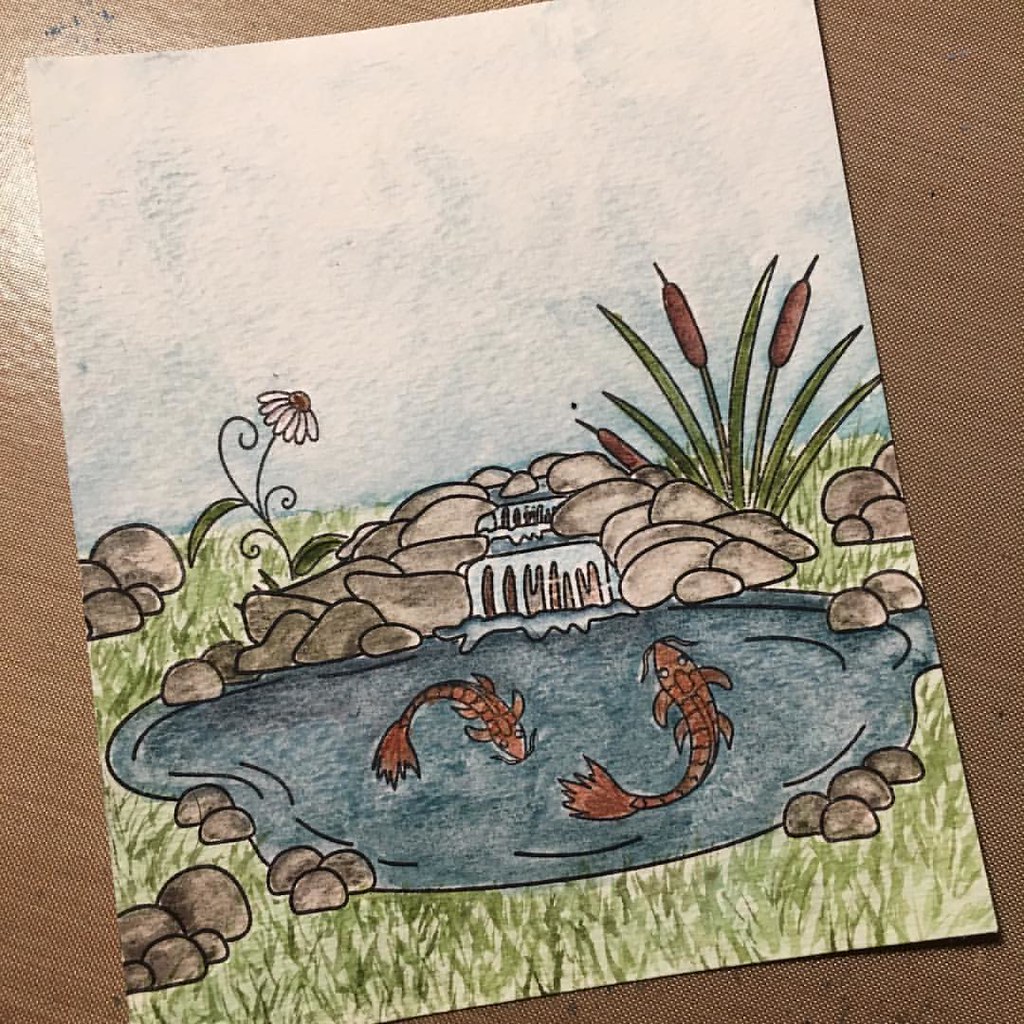This vibrant 8x10 watercolor painting vividly portrays a tranquil koi pond scene. At the foreground, a small cascading waterfall gracefully descends into the pond, which is home to two elegant koi fish, their vivid colors contrasting beautifully with the serene blue water. Encircling the pond are clusters of smooth rocks and lush grass, creating a natural and calming border.

In the background, delicate pussy willows add an element of gentle texture, while a lone daisy stands out with its cheerful presence. The artist has skillfully captured a serene sky, with soft hues of blue and white that lend a sense of peace and spaciousness to the composition.

The artwork itself is created on high-quality art paper, which rests on a simple laminate brown table, serving as a neutral backdrop that emphasizes the vivid colors and intricate details of the painting. The two-tiered waterfall structure is a central feature, guiding the viewer’s eye gently down to where the water meets the koi pond, encapsulating the essence of tranquil natural beauty in this exquisite piece.